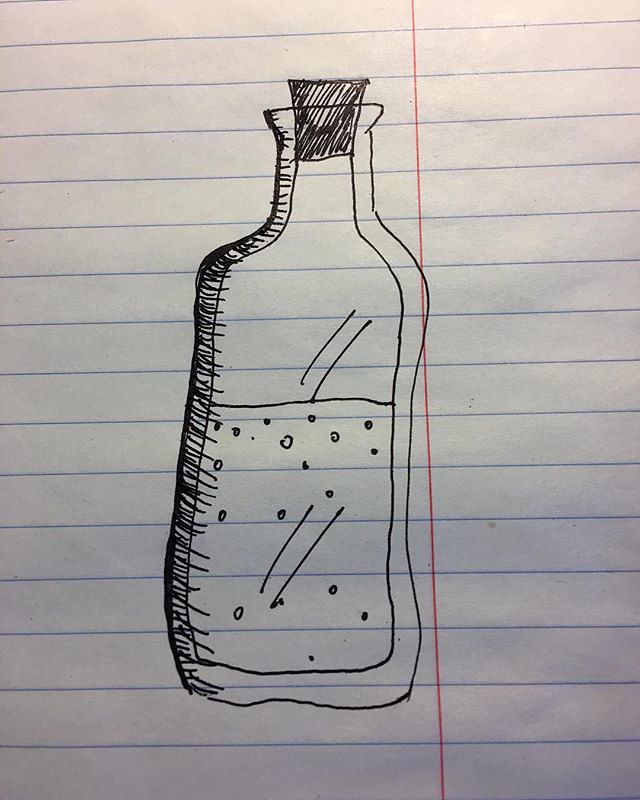This color photograph captures a black pen drawing meticulously rendered on a sheet of notebook paper, characterized by its horizontal blue-gray lines and a single vertical red margin line. The drawing depicts a bottle with exquisite detail, showcasing both the glass structure and the bottle's contents. Executed with a thin-lined black marker, the illustration features meticulous cross-hatching on the left side, suggesting shading and depth.

The artist has skillfully indicated the curvature of the glass through a parallel interior line, adding depth to the transparent material. A horizontal line demarcates the liquid inside the bottle, further detailed with small circular dots representing bubbles or particles suspended in the fluid. The reflection on the bottle is accentuated by dual lines at the top and bottom, giving the glass a realistic gleam. The cork at the top is densely shaded, adding a solid black contrast to the overall composition. This impressive and carefully crafted drawing demonstrates significant skill and attention to detail.